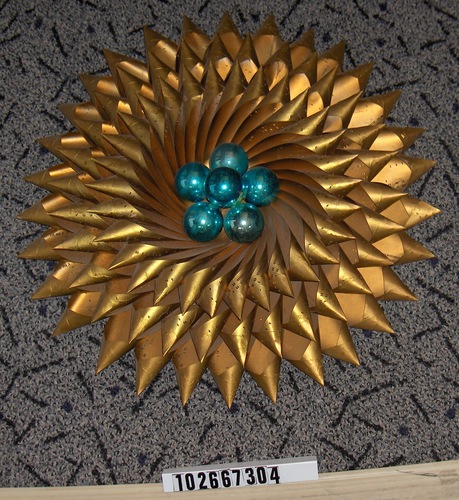This detailed photograph captures a handcrafted, abstract wall art piece resembling a sun or floral design, meticulously arranged on a gray carpet featuring a black abstract pattern. The central focus is a bronzy gold metallic structure composed of multiple layers. The outermost layer showcases approximately 32 conical, sharp-edged, pencil-tip-like spikes radiating outward, forming the base of the design. Atop this, a smaller, similarly styled circular layer adds depth and complexity. Decoratively placed in the center are six shiny turquoise balls, arranged in a star or snowflake pattern, providing a striking color contrast. Below the intricate metal artwork, a white strip with the number "102667304" is visible, possibly serving as an identification or catalog number. The overall aesthetic captures the essence of photographic representationalism, highlighting the texture and craftsmanship of the piece.